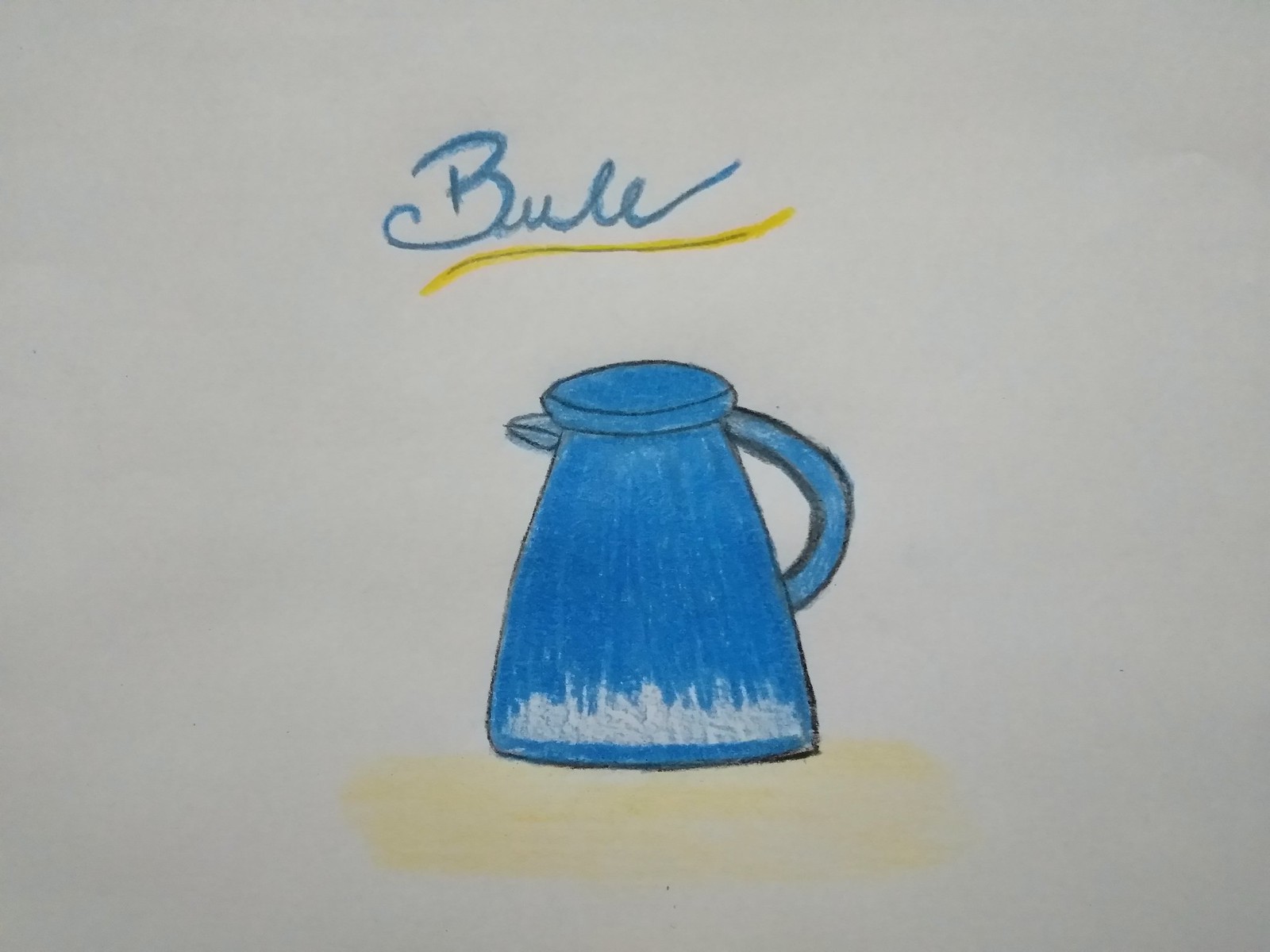This is a detailed drawing of a blue coffee pot or kettle, sketched and colored using crayon or colored pencil, on a piece of white printer paper with a noticeable texture. The coffee pot has a wide base, a handle on the right side, and a spout on the left, topped with a blue lid. The blue coloring is prominent, except for some white highlights at the bottom to give a reflective effect. Beneath the coffee pot, there is yellow shading, possibly indicating a tabletop. Above the coffee pot, the word "BULE" is written in a cursive, blue-outlined script, originally drawn in pencil. This blue script is accentuated with a decorative yellow line beneath it. The drawing is simple and straightforward, creating a contrast with the grayish-white background.